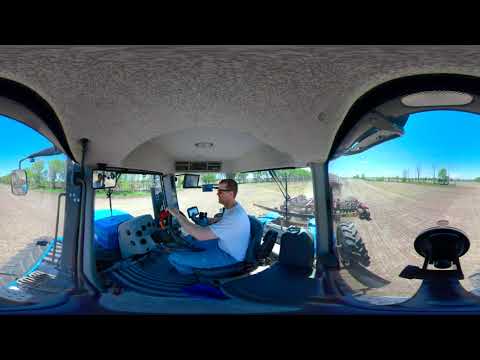The image depicts a Caucasian man with short brown hair wearing sunglasses, a white t-shirt, and blue jeans, seated in the cab of a large blue combine tractor. The photo, taken with a fisheye lens, creates a convex effect with visible bubbles around the edges. The tractor seat he is on appears to swivel, with the instrument panel and various controls in front and to the right of him. His right hand is on the steering wheel. The cab interior features black bucket seats and a tannish-white roof with an air conditioning unit above his head. Side mirrors and tractor tires are also visible. The tractor operates in a dry, dusty field, where plowing or disking equipment is being used, as indicated by the farm implements visible behind the tractor. The surrounding environment includes a bright blue sky, distant green bushes, and trees along the field's edge.